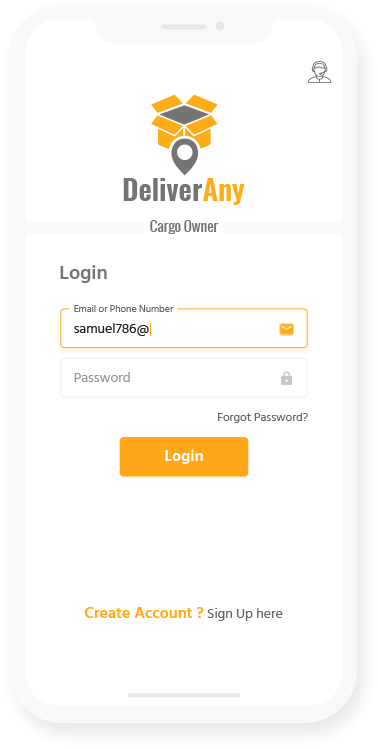The image features a user interface screen with a light gray background and rounded corners. At the top, there's an illegible word due to its small size. The upper right corner depicts an icon of a person wearing headphones with a microphone, likely signifying customer support. 

Centrally, a yellow box with a gray interior and an upside-down teardrop containing the phrase "Deliver Any" draws attention. Below this, a light gray line carries the label "Cargo Owner," followed by a white background section.

In the login section, there's a rectangle outlined in orange labeled "Email or Phone Number," which contains a placeholder and an email address. Adjacent to it is a yellow rectangle with an arrow pointing downward. A gray-outlined box marked "Password" includes a gray lock icon on its right side.

Below, the interface offers a "Forget Password?" link, followed by an orange "Log In" button. Further down, a prompt in orange reads "Create Account?" with "Sign Up Here" in black text next to it. The image concludes with a gray horizontal line at the bottom.